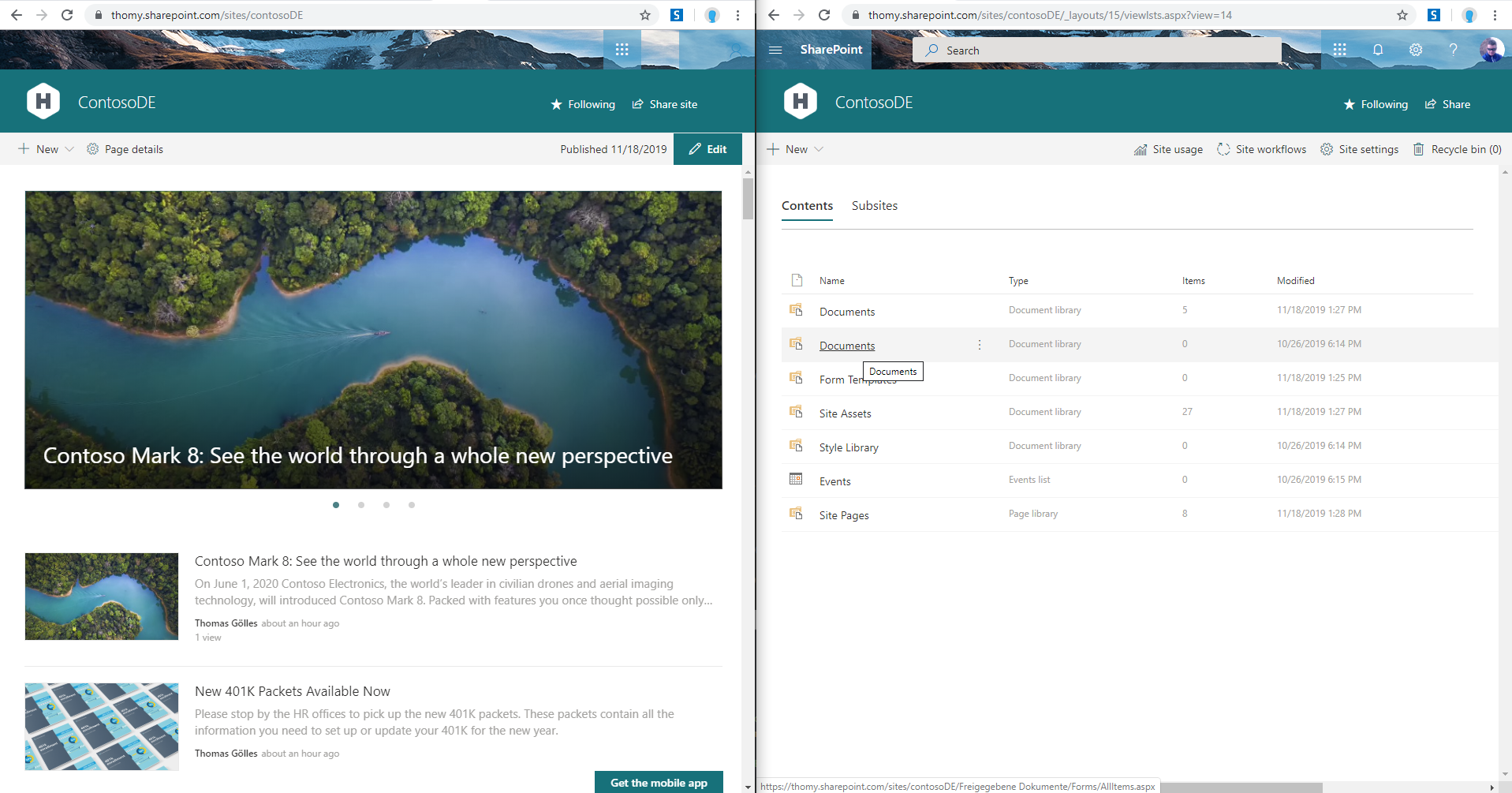Two screenshots display a website with a consistent address. Each screenshot has a striking dark green header featuring the logo "Comasco" or possibly "Contasso" with distinctive caps: "D-E-C-O-M-O-S-C-O" and "C-O-N-T-O-S-S-O-D-E."

The first screenshot captures a page with a serene image of a lake beside the "Contasso Mark 8" tagline, which invites viewers to "see the world through a whole new perspective." Below this tagline, a series of four dots is displayed, with the first dot shaded in dark gray, indicating it is the active section.

Adjacent to the featured image of the lake, there is an article layout accompanied by another picture. This image consists of a pattern formed by various shades of blue rectangles, ranging from light to dark blue, contributing to a visually engaging and informative layout.

The second screenshot retains the green header with "Comasco" or "DECOMOSODE." A profile picture is visible in the top right corner. The interface includes a 'new' button marked with a plus sign, alongside options labeled "contacts" and "contents," with "contents" prominently underlined, indicating the active section.